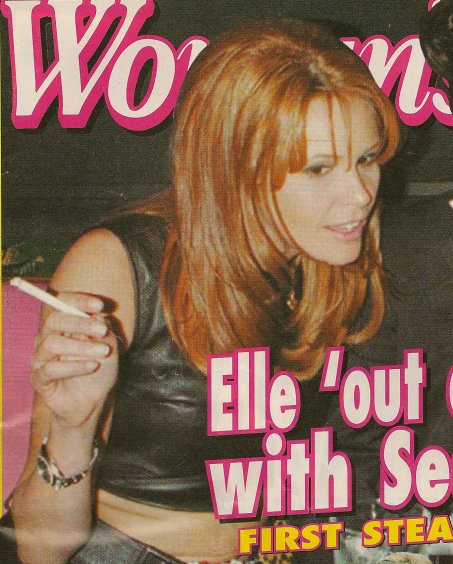The image features a striking photograph of a woman, likely Elle Macpherson, who is positioned against a nearly black background, suggesting a magazine cover. She has vibrant, long, straight red hair falling to her chest, and she is wearing a black leather sleeveless tank top that exposes her midriff, paired with leather pants. She holds a lit cigarette in her right hand, with her elbow bent upwards, and a silver metallic watch adorns her right wrist. The photograph is shot vertically and is likely rectangular in shape.

The background showcases partially obscured text that appears to be the name of the magazine, with fragments of white and pink letters visible, potentially spelling "WO" and "N" of a word resembling "woman." Below her face, more fragmented text spells "L out with C" and "StEA" in white letters with pink and yellow outlines, though the words are not fully legible due to being cut off by her positioning. The overall composition of the image is indicative of a high-fashion editorial design.